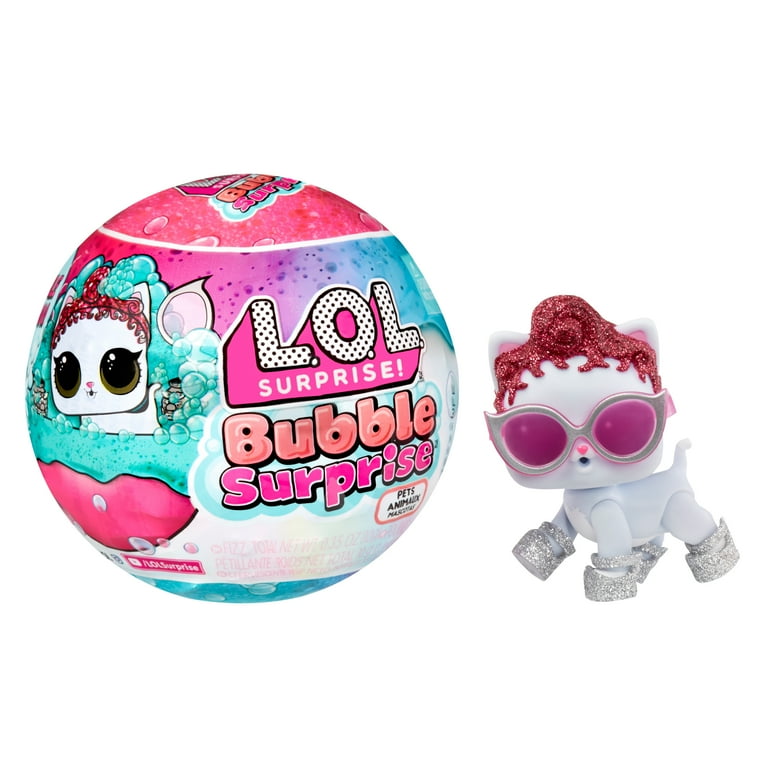The image depicts a detailed scene centered around an "LOL Surprise! Bubble Surprise" toy set. On the left side, there is a colorful, spherical package labeled "LOL Surprise" with black and white polka-dotted lettering and a pink backdrop for the word "Bubble" and a blue backdrop for "Surprise." The text appears to have a 3D effect, giving it a dynamic look. The package also features an image of a small white dog, which looks like it’s part of the toy collection.

On the right side of the image, the unboxed toy is prominently displayed. It appears to be a combination of a stylish cat and dog, featuring playful, child-friendly details. The toy is accessorized with vibrant sunglasses, silver shoes, and something red adorning its head, possibly mimicking hair or a hat. The overall aesthetic, with its vivid colors and whimsical design, suggests it is intended for children, though it might also serve as a collectible for some adults. The scene evokes a sense of playful adventure, hinting that both the toy and its packaging are meant to offer excitement and fun.